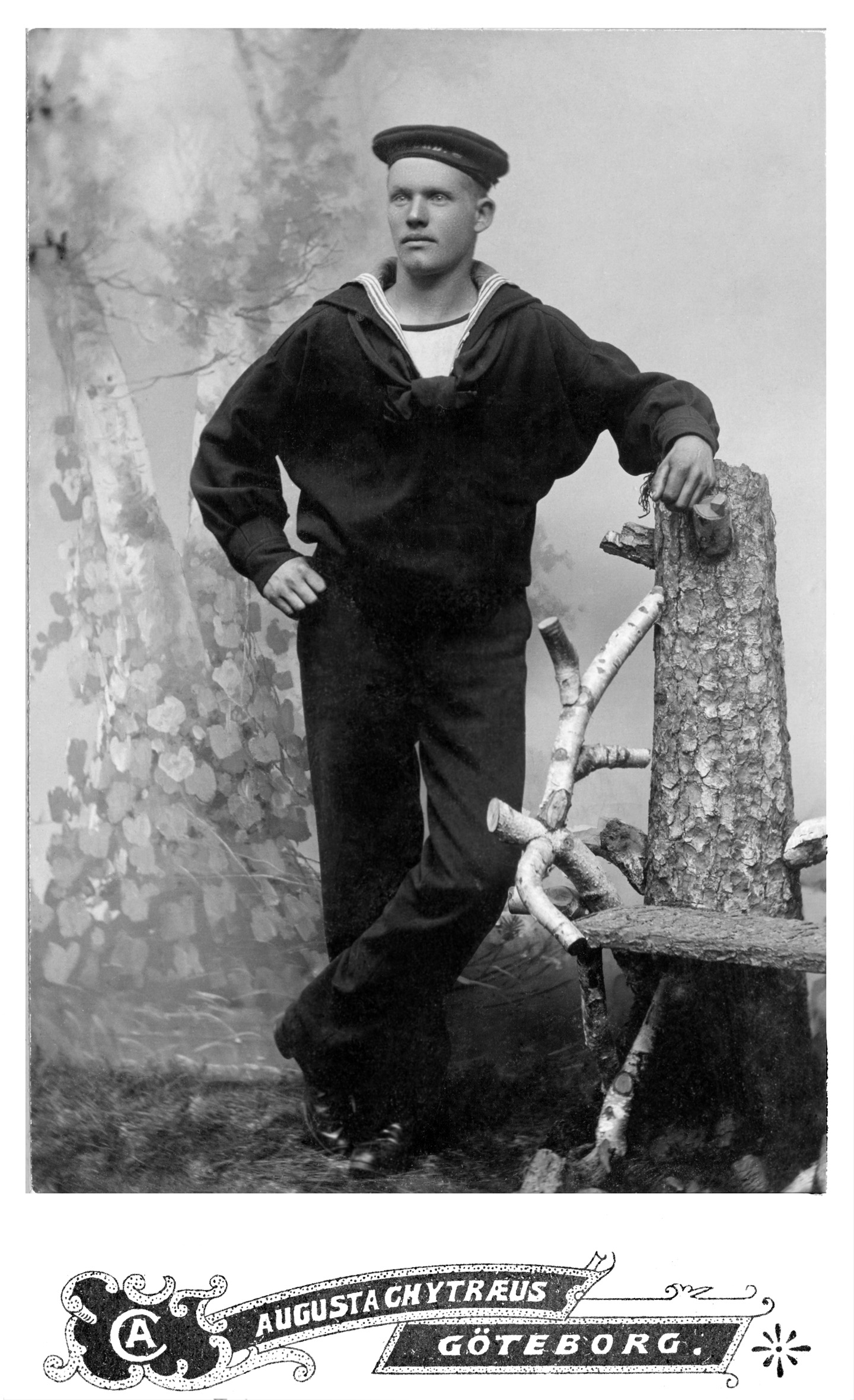This black-and-white photograph features a young man dressed in a sailor's uniform, consisting of a dark jacket with a white interior, a white shirt with a blue collar, and dark pants. He wears a sailor's cap and has pale skin. The man stands on grass, leaning his left arm against a tall tree stump while his right hand rests on his right hip. His left foot is crossed over his right, with his left leg slightly lifted. The background of the image is hazy, as if shrouded in fog, revealing only a few tree branches entwined with vines. Beneath the image, a black banner with white text reads "Augusta Titrus Gothenburg," adding a formal touch to the scene. The man's expression is blank as he gazes off into the distance, creating an enigmatic and atmospheric portrait.